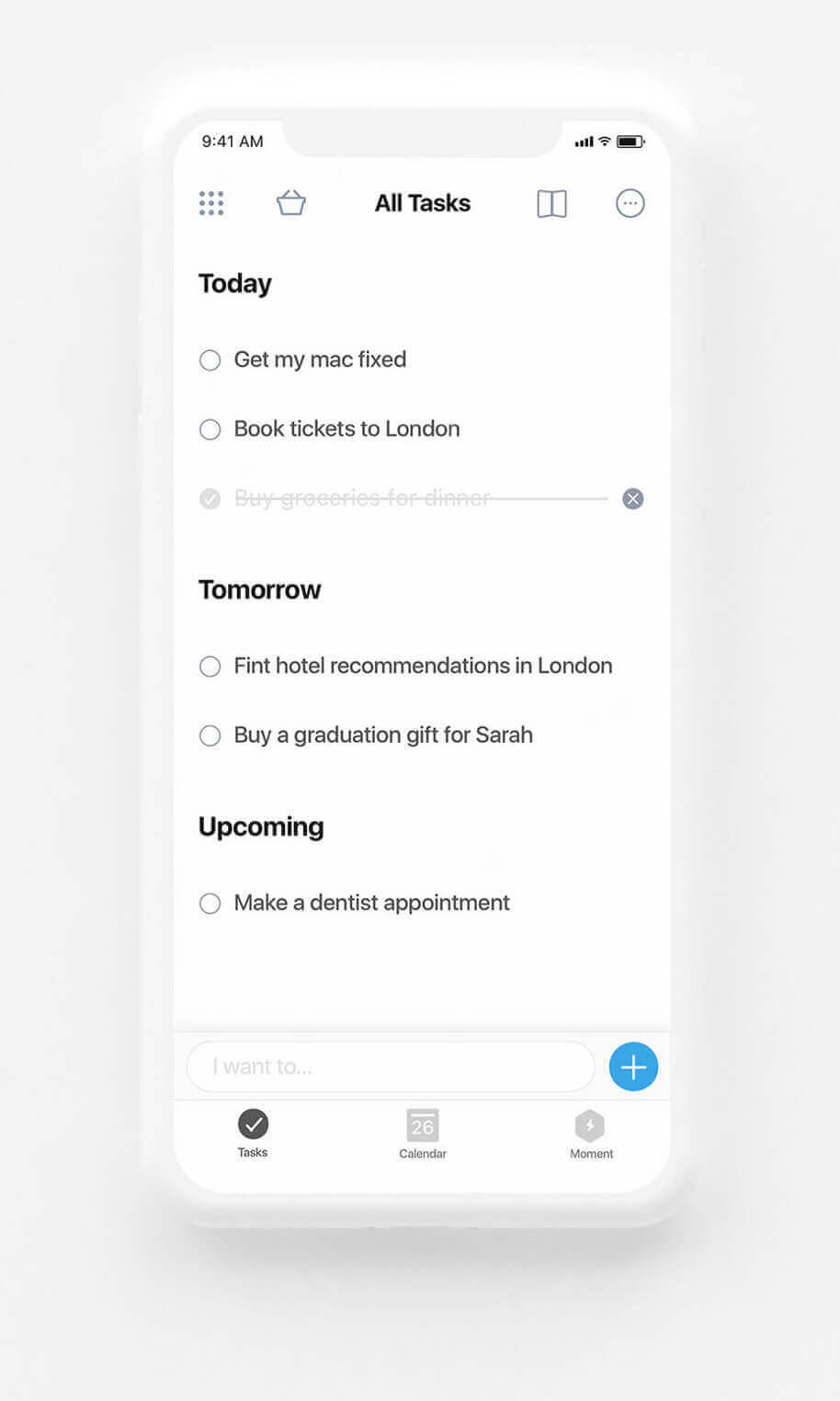The image features a screenshot from a phone, displayed against a neutral gray background. The screen capture appears centered within the image. At the very top left corner of the phone screen, the time is displayed as 9:41 AM. In the top right corner, there are indicators for full signal strength and almost full battery life.

In the top center of the screenshot, the text "All Tasks" is prominently displayed in bold letters. Flanking this text are two icons on each side. To the left, there's a grid of nine dots arranged in a 3x3 pattern, alongside an icon resembling a small pot or container. To the right, there is an icon depicting overlapping pages and another circular icon with three vertical dots in its center.

Below "All Tasks," the section is titled "Today" in bold text. Listed under this heading are three tasks. Two tasks remain unchecked: "Get my Mac fixed" and "Book tickets to London." The third task, "Buy groceries for dinner," is marked complete with a checkmark, grayed out, and struck through. An 'X' icon next to this task likely allows for its removal.

Further down, under the bold heading "Tomorrow," there are two more unchecked tasks: "Find hotel recommendations in London" and "Buy a graduation gift for Sarah." Finally, the section labeled "Upcoming" contains an unchecked task: "Make a dentist appointment."